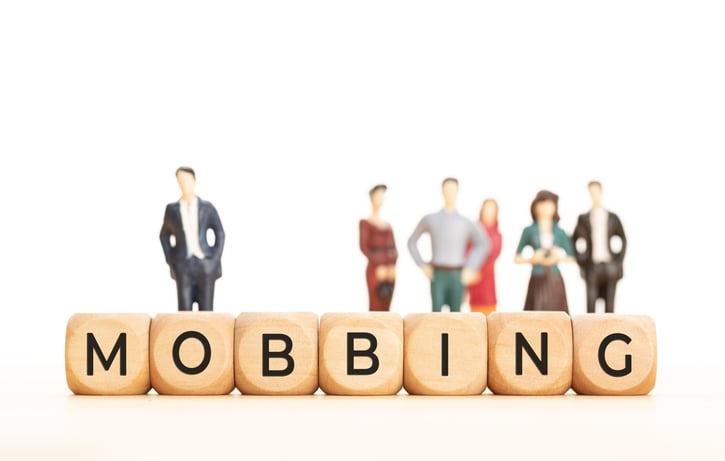In the image, we see a close-up of brown dice arranged in a line to spell out the word "M-O-B-B-I-N-G" in black letters. These dice are prominently displayed against a white background. Behind the dice, a series of blurred, cartoon-like figures are lined up, resembling action figures. On the left side behind the "O," there is a lone male figure in a black suit with a white shirt underneath. To his right, behind the other letters, are five additional figures. Starting from behind the first "B" on the right, there's a woman in a red dress, followed by a man in a gray shirt and blue pants behind the "I." Behind the second "B" is a woman in a pinkish dress. Following her and behind the "N," there's a woman with brown hair wearing a blue jacket and brown skirt. Finally, behind the "G," another male figure in a black suit can be seen. The overall scene suggests some form of social dynamic, though the exact context or message remains unclear.